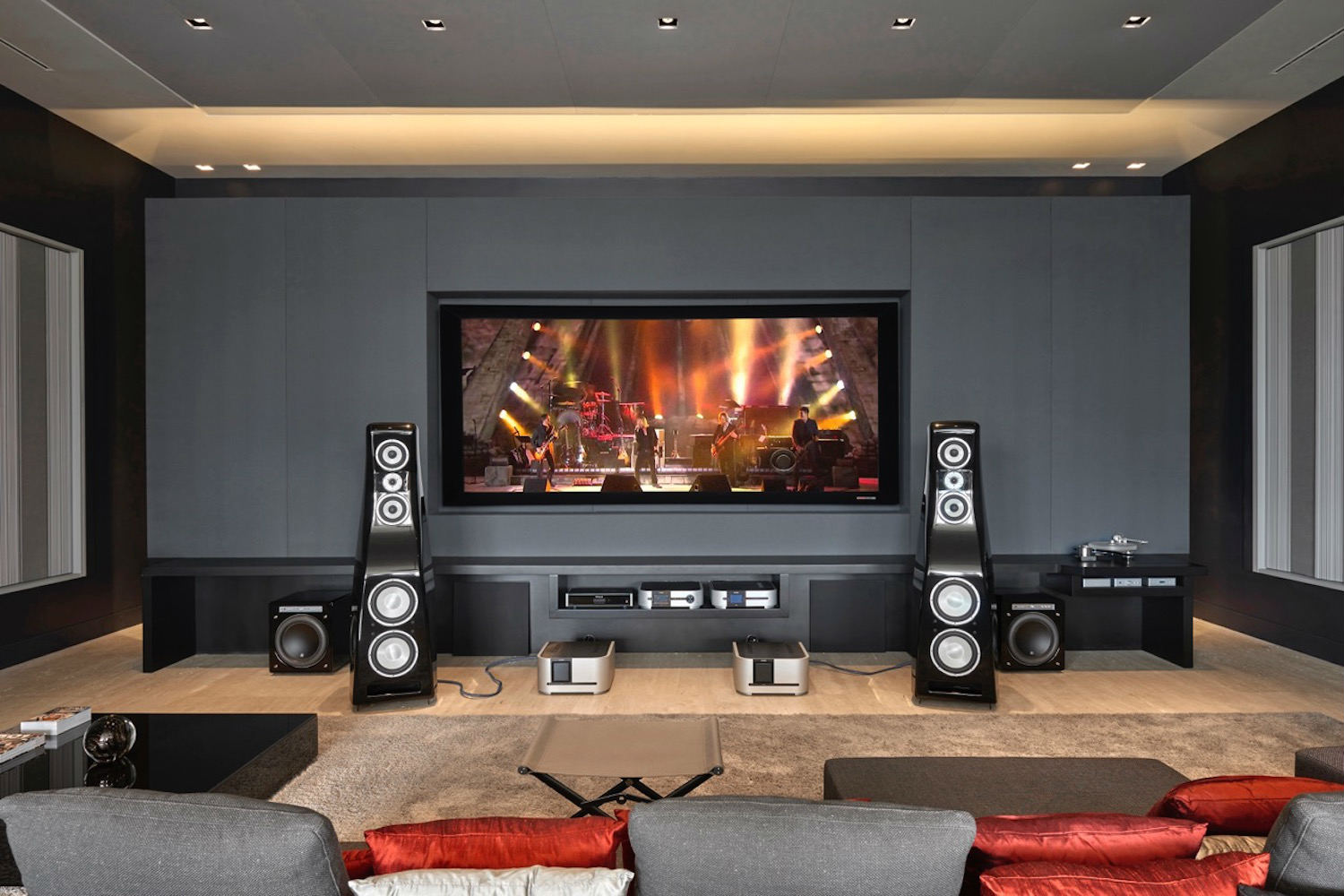This image captures a high-end home theater room with a modern and sophisticated setup. Dominating the scene is a large flat-screen TV, which is inset into a dark wall, displaying a live concert with a rock band illuminated by many lights. Flanking the TV are two substantial, modern-looking speakers, complemented by additional subwoofers on the sides and two smaller speakers positioned on the floor. Beneath the TV, a cubbyhole houses an array of DVD players, satellite receivers, and other media devices. The room itself exudes luxury, featuring gray and black walls, recessed lighting, and a beige-ish brown modern wooden floor. In the forefront, there's a sizable couch adorned with a mix of red, orange, gray, and white pillows, along with a black marble table to the left side and a folding TV tray in front of the sofa. This elegant setup unmistakably belongs to a very affluent individual.